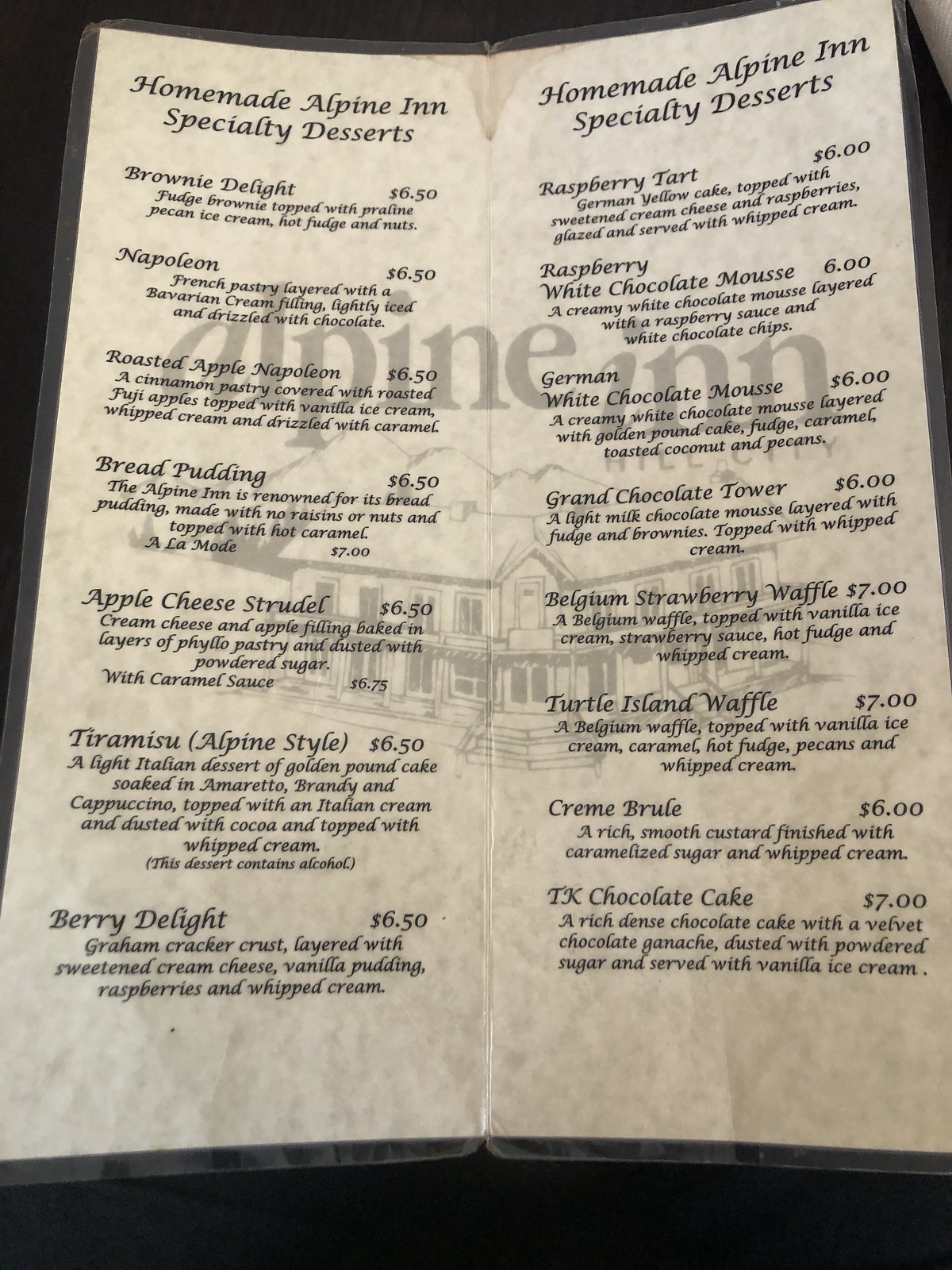This image showcases the dessert menu at Alpine Inn in Hill City. Starting from the left, the menu lists an array of homemade specialty desserts priced at $6.50 each:

- **Brownie Delight**: A rich fudge brownie topped with pecan ice cream, hot fudge, and nuts.
- **Napoleon**: A French pastry cut and layered with Bavarian cream filling, lightly iced and drizzled with chocolate.
- **Roasted Apple Napoleon**: A cinnamon pastry covered with roasted Fuji apples, topped with vanilla ice cream, whipped cream, and drizzled with caramel.

Further down, the menu highlights several other exquisite desserts:

- **Bread Pudding**: Alpine Inn’s renowned bread pudding made without raisins or nuts, topped with hot caramel a la mode. This dessert is priced individually at $7.
- **Apple Cheese Strudel**: A delightful combination of cream cheese and apple filling, baked in layers of phyllo pastry and dusted with powdered sugar. If you add caramel sauce, the price is $6.75.
- **Tiramisu**: A classic Italian dessert made with layers of coffee-soaked ladyfingers and mascarpone cheese.

On the right-hand side, the dessert selection includes:

- **Raspberry Tart**
- **Raspberry White Chocolate Mousse**
- **German White Chocolate Mousse**
- **Grand Chocolate Tower**
- **Belgian Strawberry Waffle**
- **Turtle Island Waffle**
- **Crème Brûlée**
- **TK Chocolate Cake**

Each dessert is meticulously prepared to satisfy various palates, offering a perfect ending to a meal at Alpine Inn.